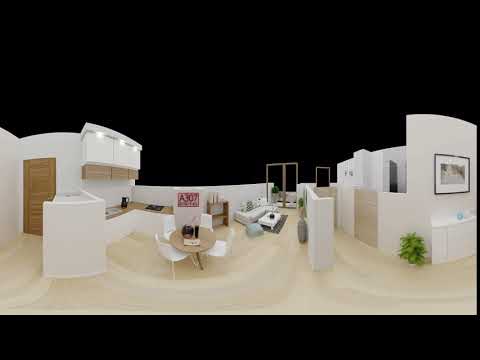The image appears to be a 360-degree mock-up of a modern home's interior, characterized by skewed perspectives and a solid black background which frames it in a square format. The left side of the image features a brown wooden door set in a white curved wall that transitions into white cabinetry with brown bottoms. Adjacent to this area, a brown L-shaped counter topped with a tan electric stovetop and possibly a black decanter can be seen, suggesting a kitchen section. In front of the counter, a wooden round table is surrounded by four white chairs.

To the right, extending from the kitchen, the space opens up into a living and dining area. Here, a white sofa adorned with throw pillows sits beside a white end table on a rug, and the floor is an ambiguous beige or light brown tile. Further along, on another curved white wall, several pictures are placed above a plant positioned on the ground. There's also mention of open doorframes that connect different sections, blending into what might resemble additional rooms possibly including a bedroom or bathroom. Despite missing ceilings and roof details, the meticulously detailed elements of this mock-up—such as the red and white poster labeled "A307", an ottoman or coffee table, and the modernistic overall look—make it a comprehensive envisioning of an interior space.